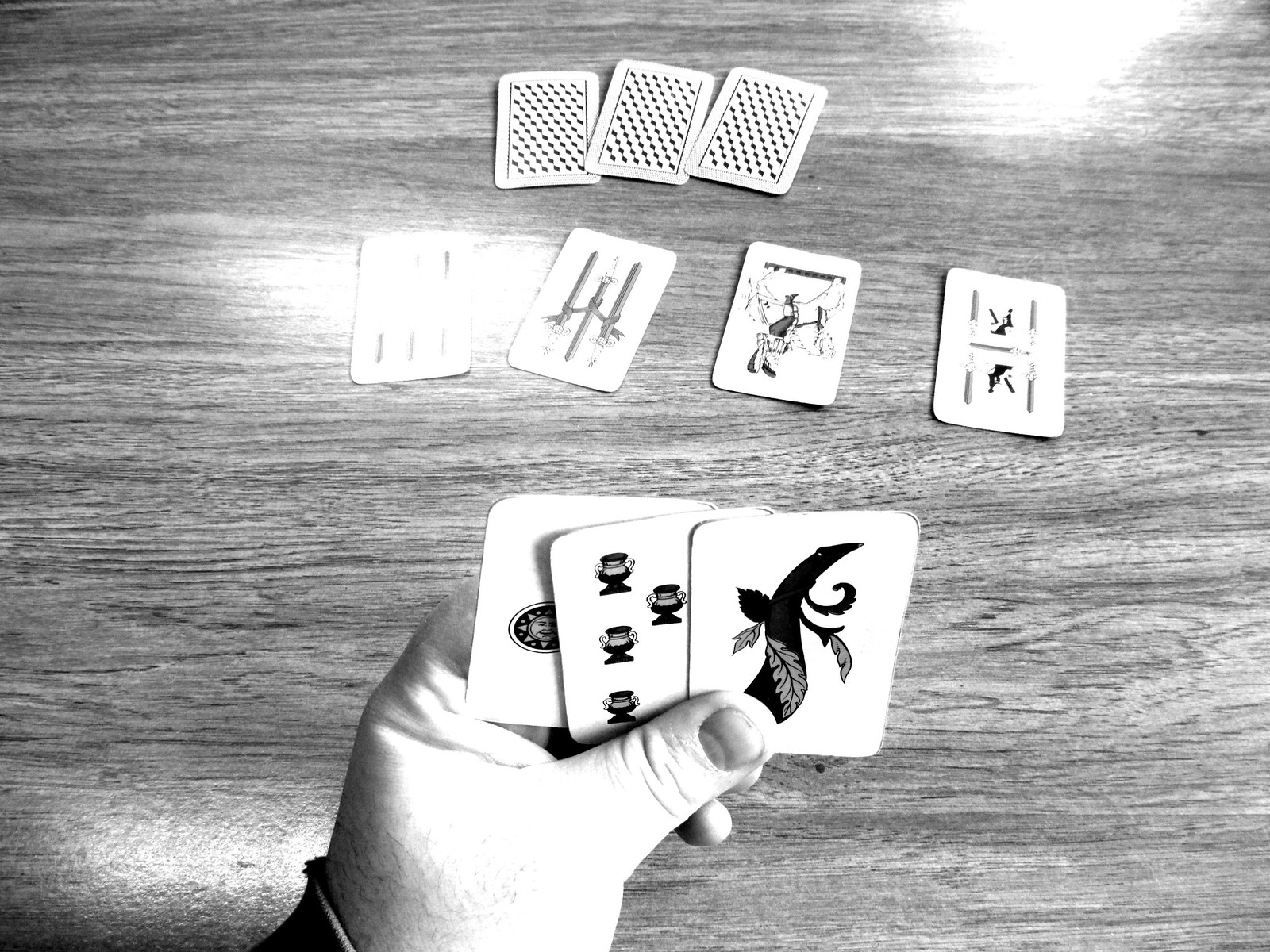In this black-and-white photograph, a person is depicted holding three distinctively illustrated cards in their left hand over a wooden table. The cards between their thumb and fingers feature unconventional images: one card shows a beanstalk, another is adorned with small lanterns, and the third displays a circle with a smiley face surrounded by triangles. On the table in front of the individual, there are four face-up cards, each bearing similarly unusual and intricate designs that are difficult to discern. Above these cards lie three additional cards placed face-down, their backs adorned with a pattern resembling a row of diamonds or small rectangular shapes. The person's hand, which is pale, is prominently positioned in the foreground, emphasizing the unique and mysterious nature of the card game being played or showcased.